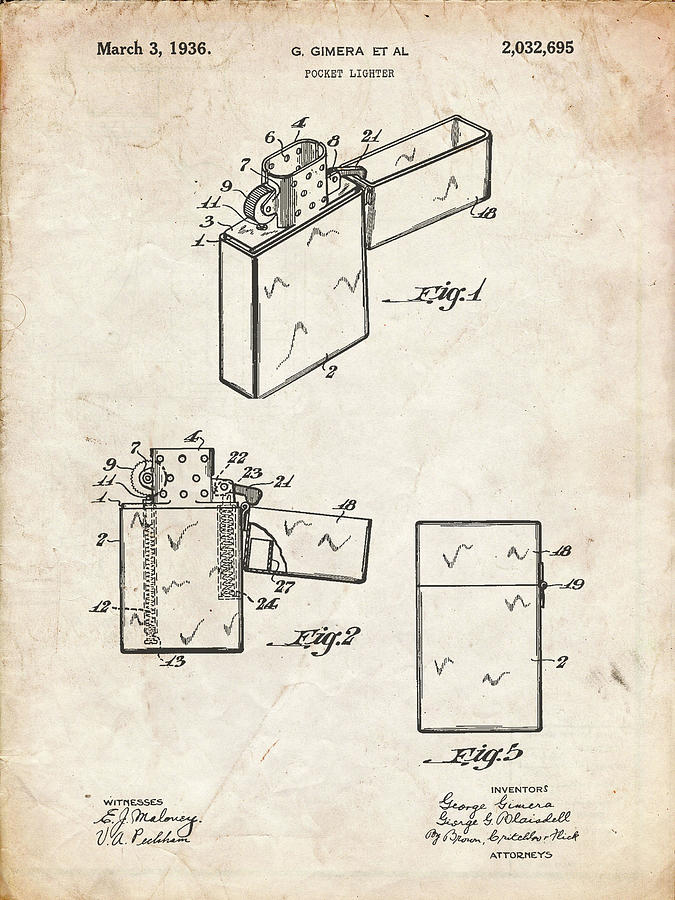This vintage off-white and light brown piece of paper from March 3rd, 1936, features a meticulously illustrated patent diagram for a Zippo-style pocket lighter. The top left of the page is marked "March 3rd, 1936," with the patent number "2,032,695" on the top right, and "G. Jemera et al." prominently displayed in the center. Below this heading, the lighter is depicted in three detailed sketches labeled Figure 1, Figure 2, and Figure 3, each identifying various parts with numbers. Figure 1 shows the lighter open, with the wheel towards the left and the open top towards the right, marked with labels pointing to different components numbered from 1 to at least 10. Figure 2, positioned to the left, displays the lighter turned sideways, again with numbered annotations. Figure 3, on the bottom right, illustrates the lighter with its lid closed, with three parts numbered and indicated. The bottom left corner lists names under "Witnesses," identified as E.J. Maloney and V.A., while the bottom right includes signatures under "Inventors" followed by "Attorneys," emphasizing the legal and collaborative nature of this documented invention. The intricate design even details the small circular holes where the flame emerges when the lid is flipped open, enhancing the technical precision of the patent illustration.